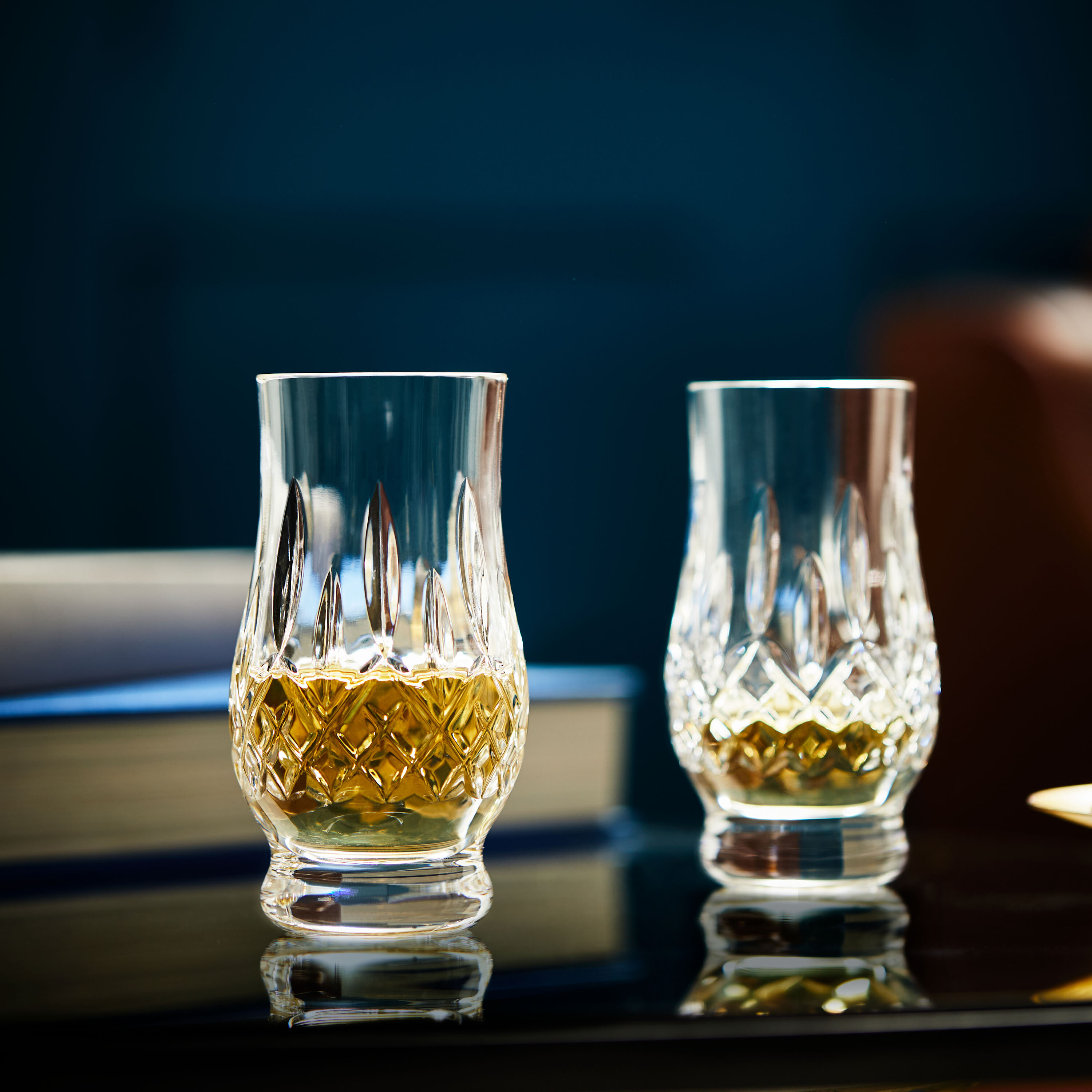The image depicts a close-up of two ornate crystal glasses, each containing a varying level of amber-colored liquid, possibly scotch or another type of alcohol. The glasses are elegantly designed with intricate cuts and patterns, reflecting the bright illumination that highlights their crystal clarity. They rest on a highly glossy, shiny black table, which mirrors their forms as well as the other items present. Behind the glass on the left, a thick book with a blue cover and white pages sits on the table, its reflection also visible on the polished surface. The background is dark and blurred, with subtle white and pink splotches and a gray stripe along the edge of the table, creating an elegantly subdued ambiance.